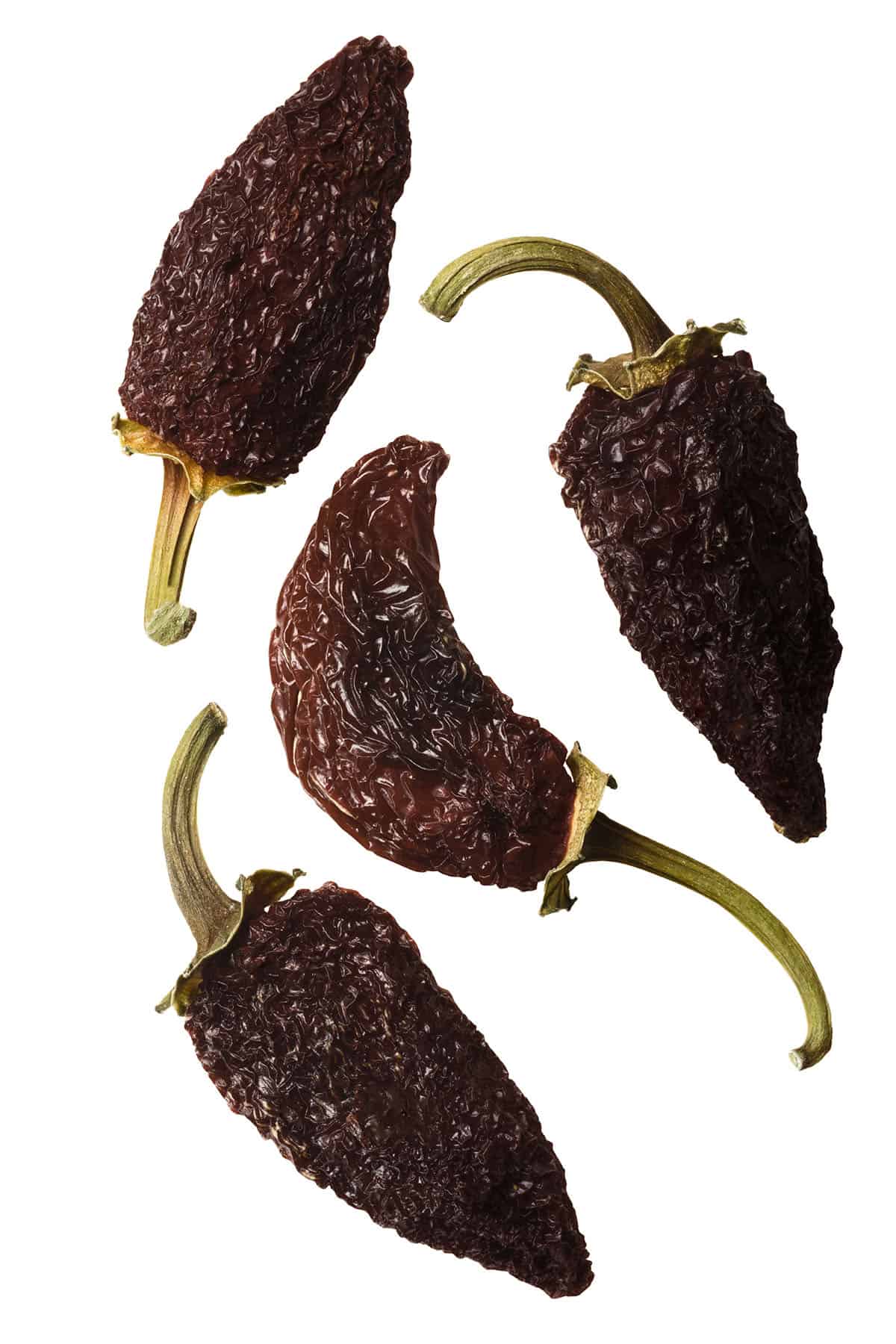In the color photograph, four dried jalapeno peppers, commonly known as chipotle, are artfully arranged against a stark white background. Each pepper has a dark brown color with a slight reddish tinge, resembling the texture and appearance of raisins due to their dryness. White specks sporadically dot the surface of these conically-shaped peppers. The pale green, curved stems on each pepper add a contrasting hue and texture. The upper left pepper, with its conical shape and curved stem, points downwards. The lower left pepper is upside down, its tip pointing to the lower right, and characterized by a similar curved stem. The middle pepper points to the upper right, and the upper right pepper points downwards, with the stem prominently positioned at the top. This detailed arrangement emphasizes both the unique and shared features of the peppers.